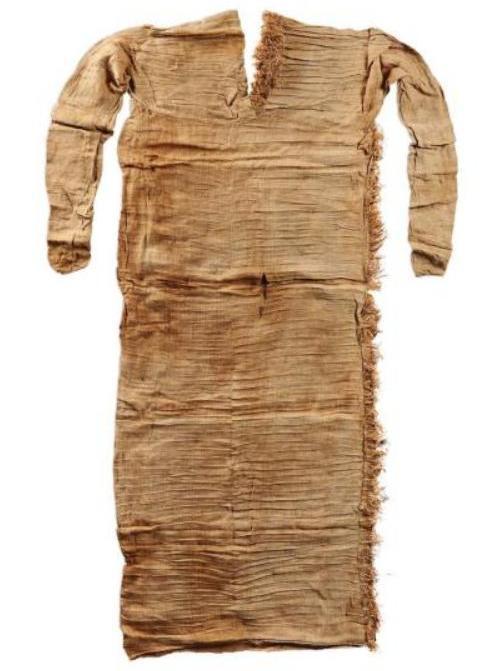This color photograph captures an angled shot of an extremely old, long-sleeved undergarment, likely a simple slip once worn by a woman. The garment, laid flat against a white background, appears to have aged significantly, its original white fabric now a tea-colored brown with darker brown areas testament to its great age. The material, possibly muslin, is notably discolored and wrinkled, especially around the collar and sleeves. The right side of the garment is particularly distressed, showing significant fraying and a noticeable split. A small, dried blood spot is visible near the waistline in the middle. The fabric appears thin and delicate, and the sleeves look as though they may have been cut off just at or below the elbows. The front of the garment features a v-shaped slit at the collarbone area. There are no sizing details or any form of writing visible on the image, emphasizing its stark simplicity and utilitarian purpose as an undergarment rather than an outer garment. The background is devoid of any people, animals, or structures, isolating the garment as the sole focus of the photograph.